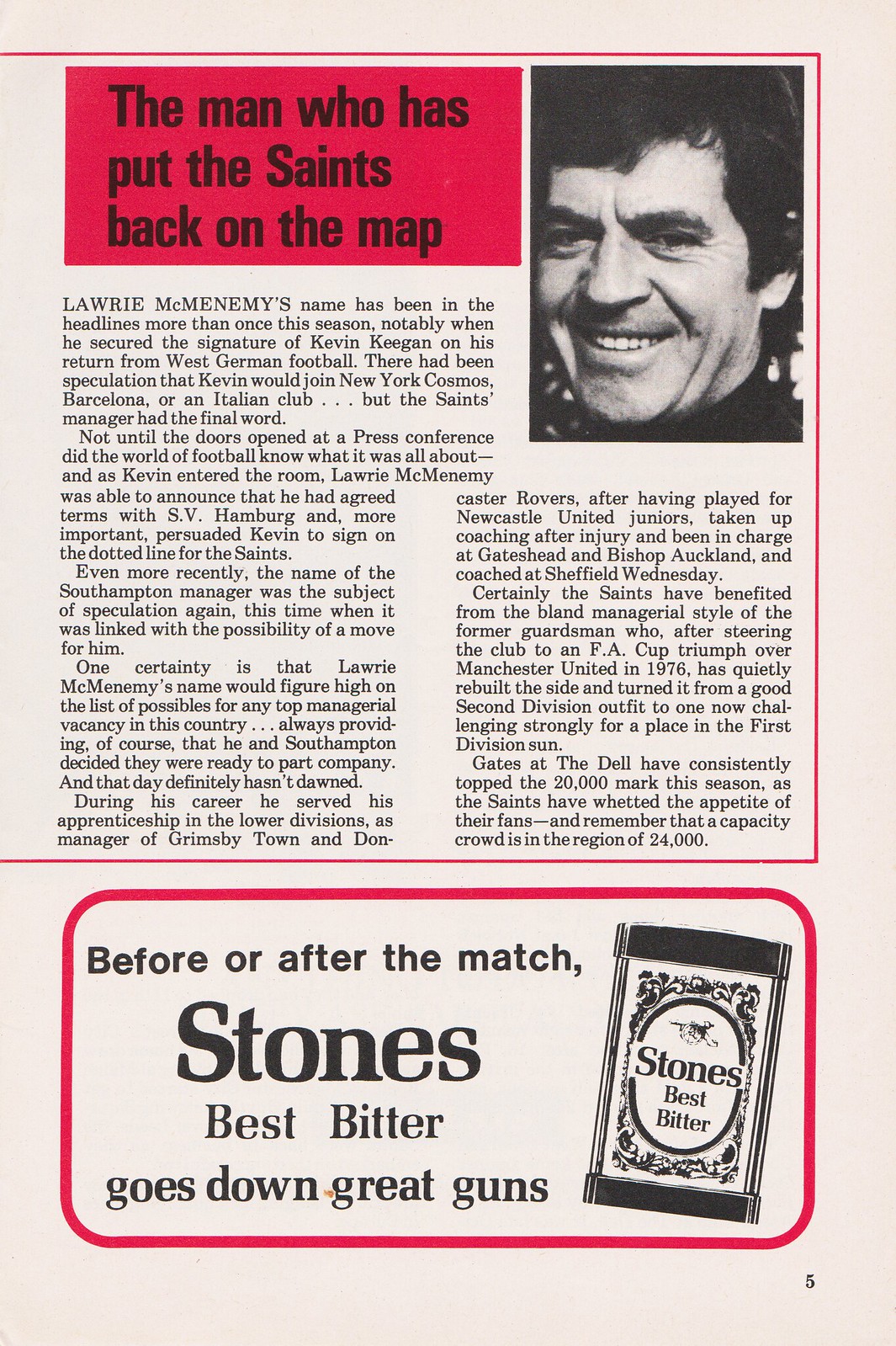The image showcases a newspaper clipping with a slightly antique, off-white color, framed by a thin red line. At the top left, in a red box with black text, it declares, "The man who has put the Saints back on the map." To the right, there's a black-and-white photo of a smiling man with medium-length, wavy black hair, possibly sporting a faint mustache and wearing a dark top. His ears are partially covered by his hair. 

The article discusses Laurie McMenemy, whose name has frequently appeared in the headlines this season, notably for securing Kevin Keegan's signature upon his return from West German football. Although there was speculation about Keegan joining New York Cosmos, Barcelona, or an Italian club, the Saints manager, McMenemy, had the final word.

Below the article, there is an advertisement framed in a red-lined rectangle, stating, "Before or after the match, Stone's Best Bidder goes down great guns," accompanied by an illustration of a tin with the same branding. This clipping is marked as page five of the publication.